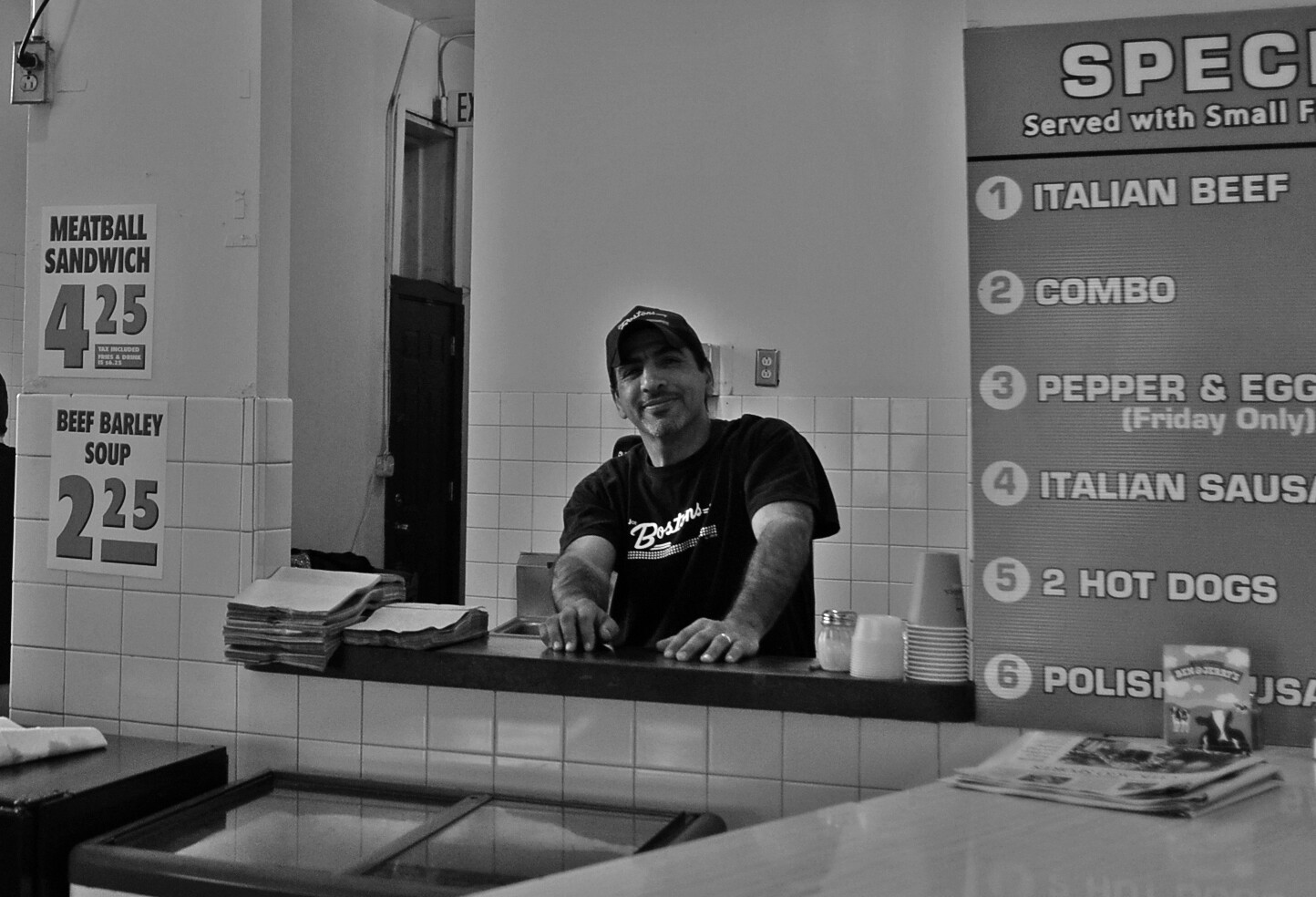This black-and-white image depicts a man standing behind a counter in what appears to be a restaurant. The man, dressed in a dark t-shirt and a cap, is smiling with his head slightly tilted counterclockwise. He has both hands resting on the counter, which is part of a cutout section of a wall. 

To the left of the man, attached to the wall, is a sign listing "Meatball Sandwich $4.25" and "Beef Barley Soup $2.25." The right side of the counter features a stack of cups and smaller containers, along with a partially visible menu sign. The menu lists various items, beginning with "served with small," followed by "1. Italian Beef," "2. Combo," "3. Pepper and Egg," "4. Italian Sausage," "5. Two Hot Dogs," and "6. Polish." The top of the sign shows the letters "S-P-E-C" and a black line beneath "served with small."

On the counter in front of the man, there is a stack of papers on the left side. Near the bottom right of the image, a Ben & Jerry's advertisement is visible along with a newspaper on another counter. Towards the lower left, the edge of a freezer case can be seen, and further left, there appears to be a mini refrigerator.